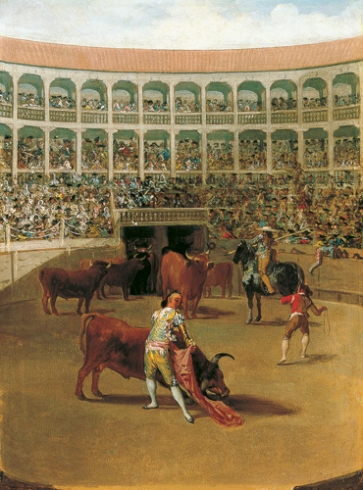This vivid painting portrays a dramatic bullfight set within a bustling, circular coliseum. Dominating the foreground, a fierce bull lunges toward a matador, who skillfully maneuvers a red cape to captivate the beast. Nearby, a mounted man on a black horse wields a staff in a defensive posture. Scattered across the arena are several calmer bulls, adding to the chaotic yet orchestrated scene. 

The ground within the ring is a dusty brown, setting a stark contrast against the structured tiers of spectators. The stands are densely packed, comprising three levels: the lowest is open seating, followed by two more levels under elegant arches supported by stone pillars, giving the area a classical, coliseum-like appearance. Above the arches, a roofline hints at a light peach or mauve color, between which strips of blue sky peek through, dotted with clouds, suggesting a pleasant day. This rich composition captures the drama and intensity of the bullfighting spectacle against the grandeur of a historical arena teeming with anticipation and energy.